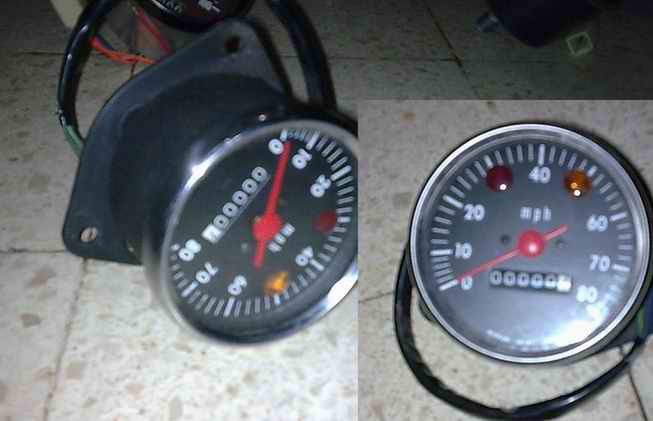The larger image showcases a rugged tile floor composed of large, stone-like tiles often found in garages and workshops. Positioned upside down on this floor is an odometer-like device with a prominent red handle and a pair of indicator lights—one red and one yellow—situated at the bottom of the picture due to the orientation. The gauge on this instrument ranges from 0 to 80, suggesting it might belong to a smaller vehicle, like a scooter, as opposed to a car. The odometer reads 0, indicating it may be newly installed. The back of this apparatus is square-shaped with two visible holes and several wires extending from it. The smaller, superimposed image offers a closer view of the device, shown right side up. Although minor light glare obscures the bottom-right corner, the detailed focus provides a clearer perspective of the instrument’s features and its pristine, unused condition.